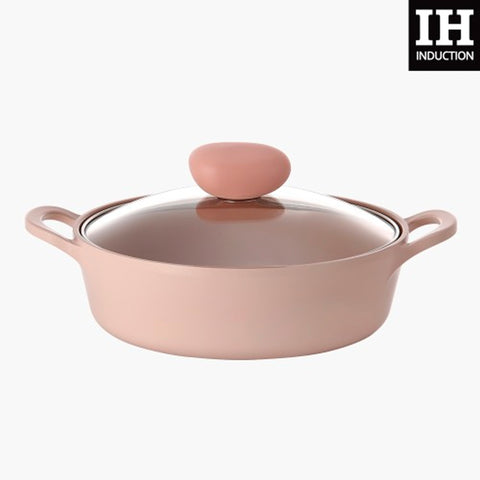This close-up photograph captures a medium-sized, light mauve pink frying pan with a glass lid. The pan features two small, standard side handles, designed for easy handling. The lid boasts an adorably large, egg-shaped pink knob with a wide top and a narrower bottom, making it convenient to grasp. The photograph’s backdrop is predominantly white, except for the upper right-hand corner, where a black square prominently displays the white capital letters "IH" with "Induction" beneath them. The pan is positioned about halfway up from the bottom of the image, and the glass lid reflects light, adding a touch of elegance.